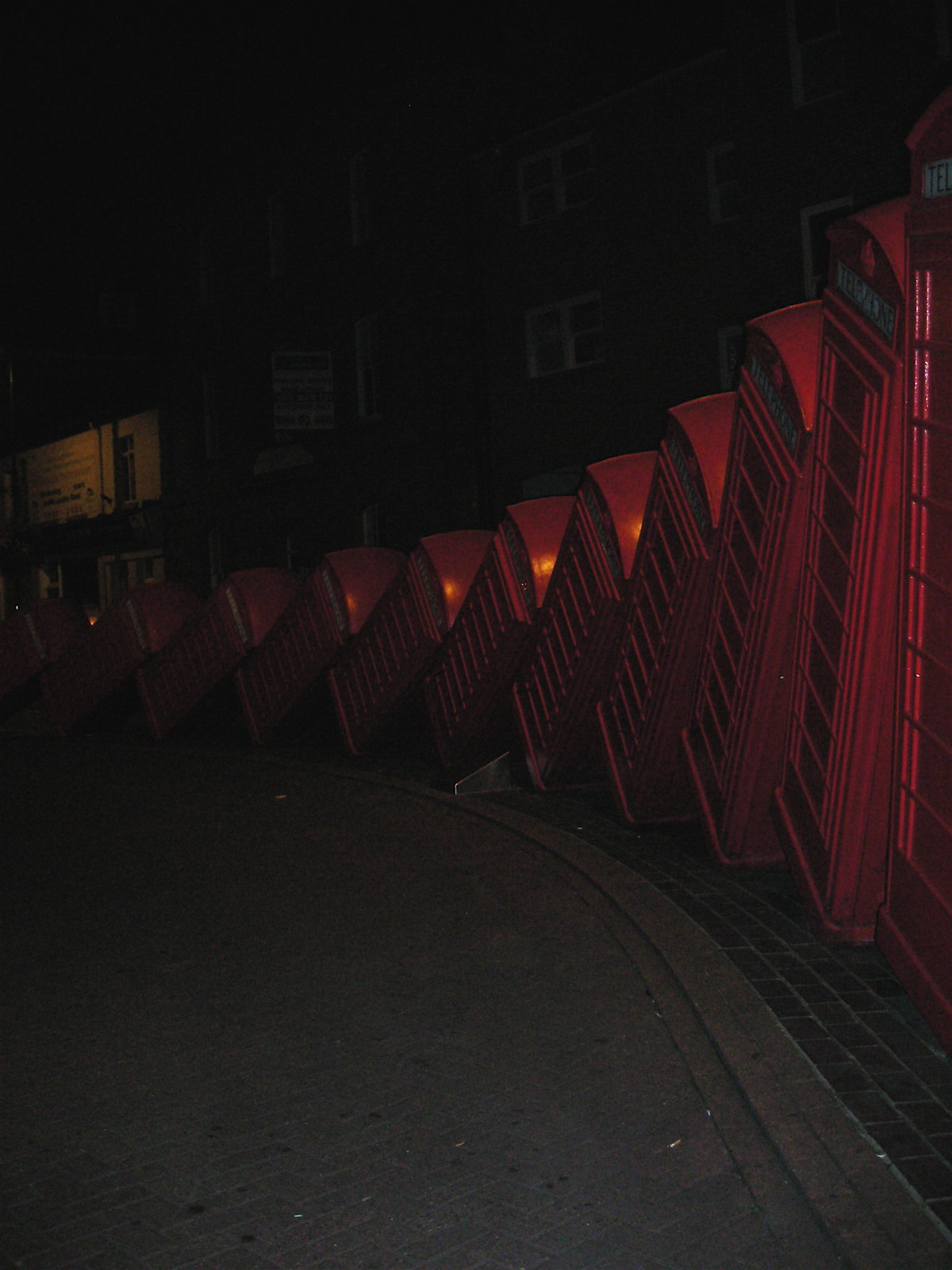The image depicts a dimly-lit, nighttime street scene where three red telephone booths are visibly leaning to the right, creating a domino effect as if they have been toppled over. Each booth, originally standing upright side-by-side, features a door with vertically arranged bars from top to bottom, and a white rectangular sign with black text reading "telephone" at the top. The booths are situated on brick tiling, with a stone road seen on the left side of the image. The faint illumination reveals the booths' windows and highlights a slightly visible building in the background, enhancing the overall dark and eerie atmosphere. The street appears to have curved walls lined with bricks on the outer edge and cement in the center, with very dim triangular light sources casting minimal light on the scene.